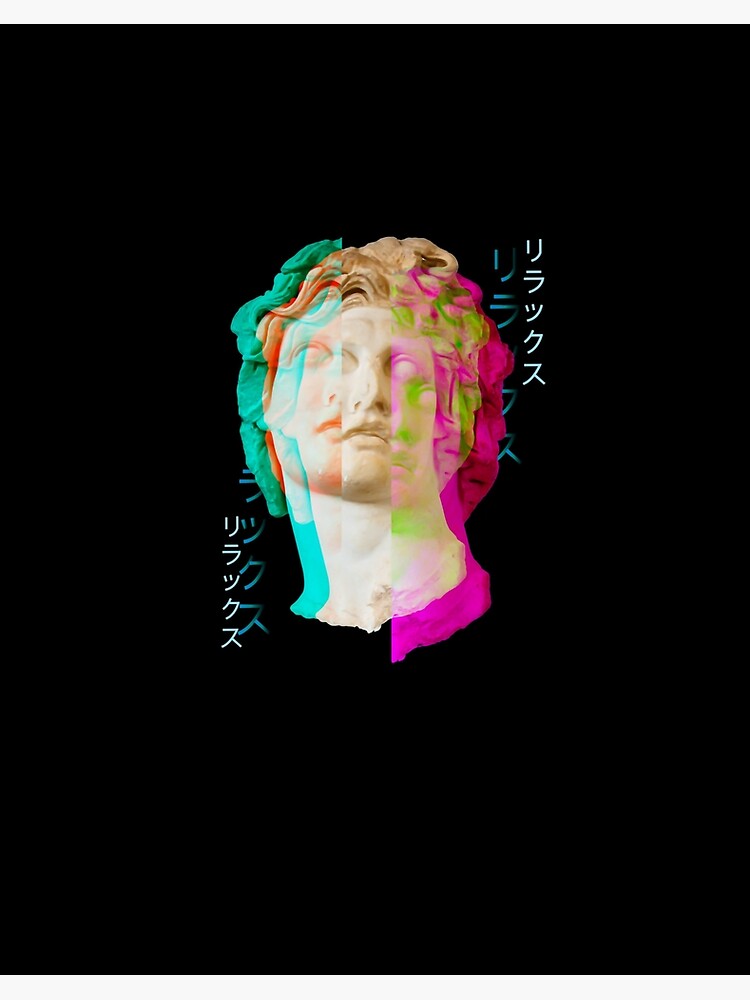In the center of the image, against a stark black background, is a marble-like statue of a head, capturing only the area from the top of the curly hair down to the bottom of the neck. This head is artistically distorted, as if multiple overlapping versions of it are present, creating a doubled or tripled appearance. The central head features brown hair, while adjacent versions on both the left and right display various hues: the left side shows hair with blue, orange, and green highlights, while the right side reveals repetitive features like three sets of lips and three eyes, but only two noses, with pink and green accents overlaying the hair and face. Surrounding the statue are Japanese or Chinese characters, placed on the lower left, upper right, and bottom left of the image. This intricate amalgamation of colors and forms, combined with the textual elements, gives the image a cohesive design reminiscent of an album cover.